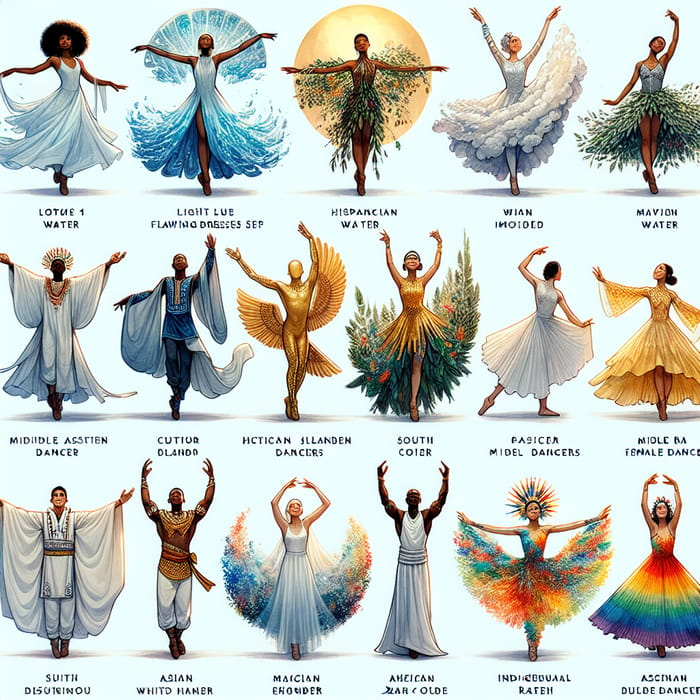This is a vibrant, color-illustrated chart featuring fifteen figures arranged across three rows—five in the top row and six each in the middle and bottom rows. These figures represent a diverse collection of individuals in various dance poses, captured in the midst of ceremonial or cultural dances. They are depicted in elaborate, flowing costumes that appear to reflect different cultures and styles, some with arms extended holding their skirts, others with arms raised, accentuating their graceful movements.

The chart includes short inscriptions beneath each figure, written in black capital letters. While some of these inscriptions are in English, others are in a foreign language, making them challenging to decipher. For example, the top left figure, a dark-skinned woman with an afro, wears a flowing white dress with spaghetti straps. The text below her reads "LOTUE, ONE WATER," likely indicating her dance style or cultural background. Adjacent to her is another dark-skinned woman with an outstretched blue dress that mimics the appearance of flowing water and waves, adding a dynamic element to the image.

Across the chart, the dancers wear an array of colorful, intricate costumes—from long, flowing dresses to ankle-length skirts and even robes adorned with vibrant designs such as peacock feathers and rainbow patterns. These attires suggest a blend of cultural influences, with elements that could be linked to Hispanic, Middle Eastern, and possibly Indian traditions. Despite the varying poses and outfits, a unifying theme of ceremonial dance positions and the beauty of diverse cultures is evident throughout the illustration.